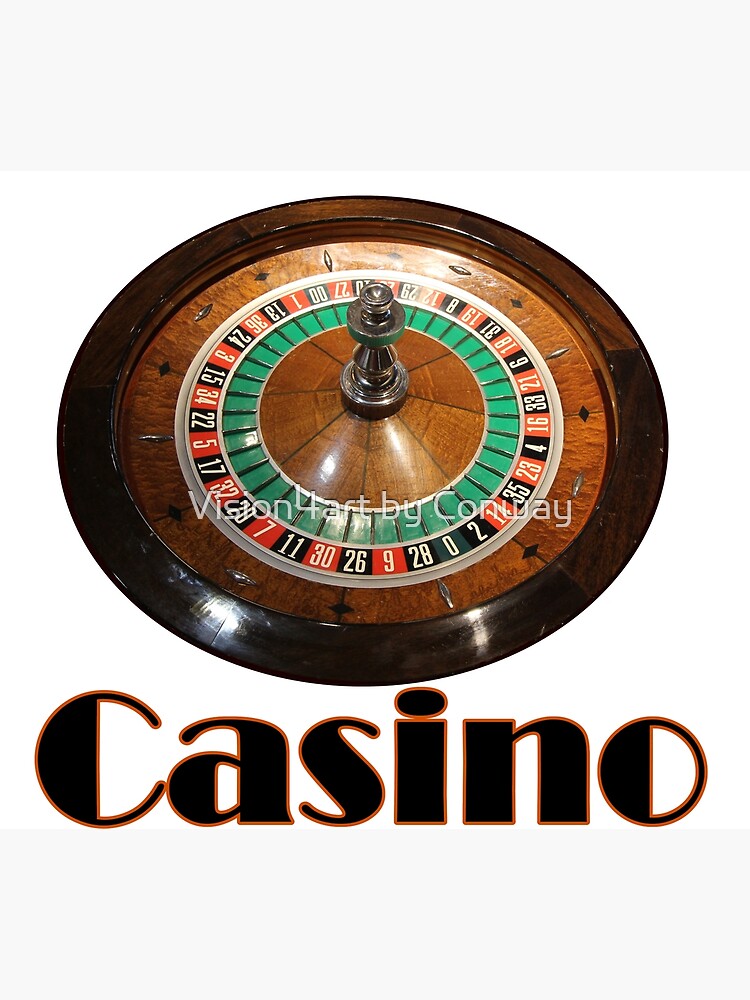This photograph features a detailed overhead view of an ornate roulette wheel set against a completely white background. The wheel is prominently centered and showcases intricate craftsmanship, with its outer rim and base made of rich, dark wood. Just inside the outer wooden rim, a circle of alternating red and black numbered compartments encircles the wheel, typical of roulette games. Further within, there's a green circle segmented by black lines, leading to a smaller central circle of the same dark wood. Rising from the center is what appears to be a brass or silver pedestal, resembling a chess piece, possibly the spinner for the wheel.

The image includes two gray boxes at the top, one directly above the roulette wheel and another positioned beneath it. Across the top arc of the wheel, faint white text reads "Vision for Art by Conway." Below the wheel, in bold black letters with a wooden outline, the word "Casino" is emblazoned. The absence of roulette balls and the inclusion of ornate details like inlaid metal or gemstones around the numbering hint that this image might serve as an advertisement or artistic representation of a roulette game.